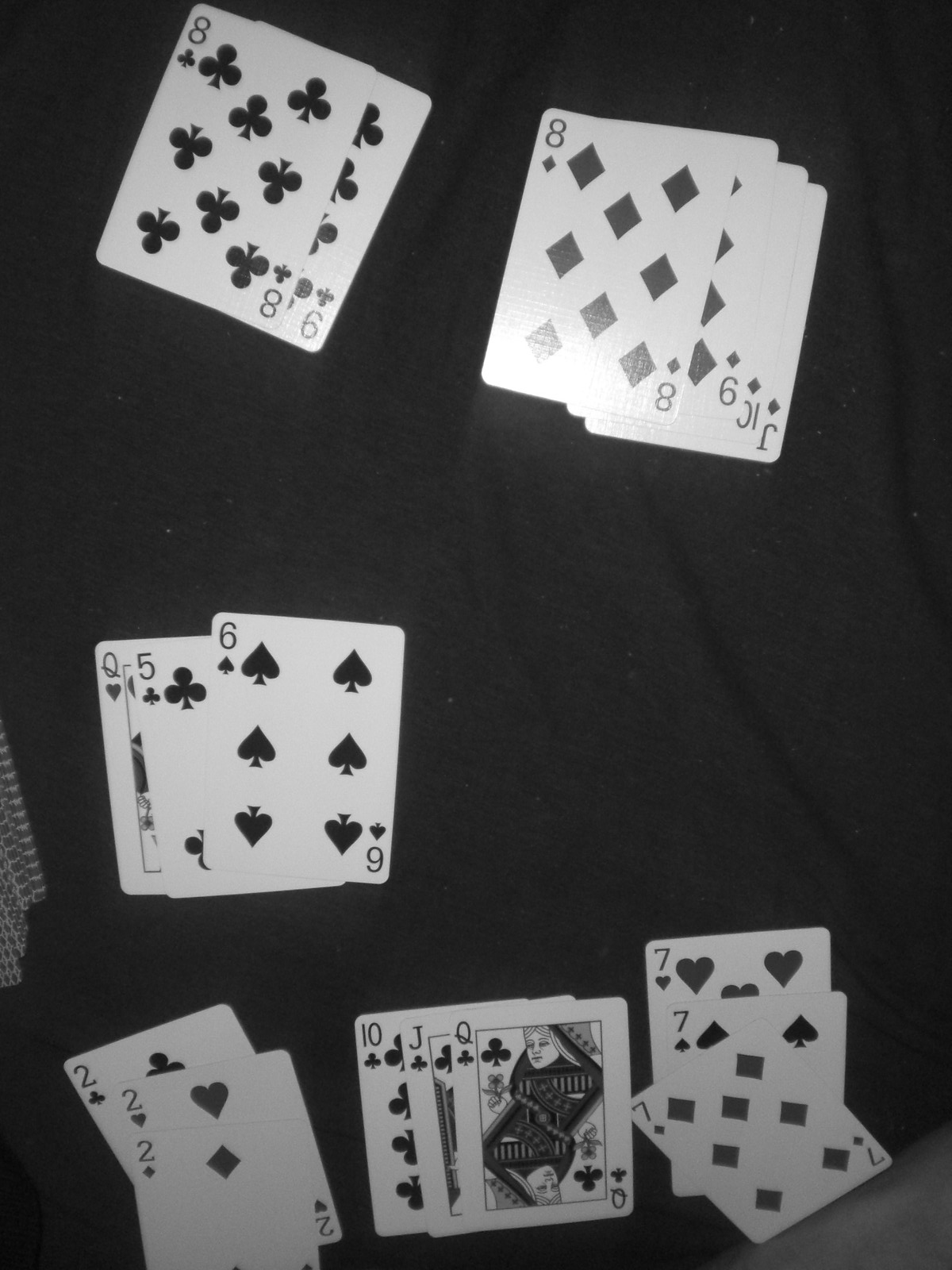This black-and-white photograph features six small stacks of playing cards arranged on a black fabric surface. The fabric showcases subtle wrinkles and tiny white or gray specks, likely indicative of dust particles. 

At the top of the image, two stacks of cards are spread out and overlapping. The stack in the upper left corner reveals two cards, both the eight of clubs. To the right, an overlapping sequence comprises the eight, nine, ten, and jack of diamonds. 

In the center of the photograph, another set of three overlapping cards can be seen: the queen of hearts, the five of clubs, and the six of spades. Below this central stack are three additional overlapping stacks. The leftmost stack consists of the two of clubs, two of hearts, and two of diamonds, while the middle stack displays the ten, jack, and queen of clubs. The rightmost stack features three sevens from different suits: hearts, spades, and diamonds.

A faint reflection of light is noticeable on the upper right stack comprising the eight, nine, ten, and jack of diamonds, adding a subtle highlight to the otherwise monochromatic composition.